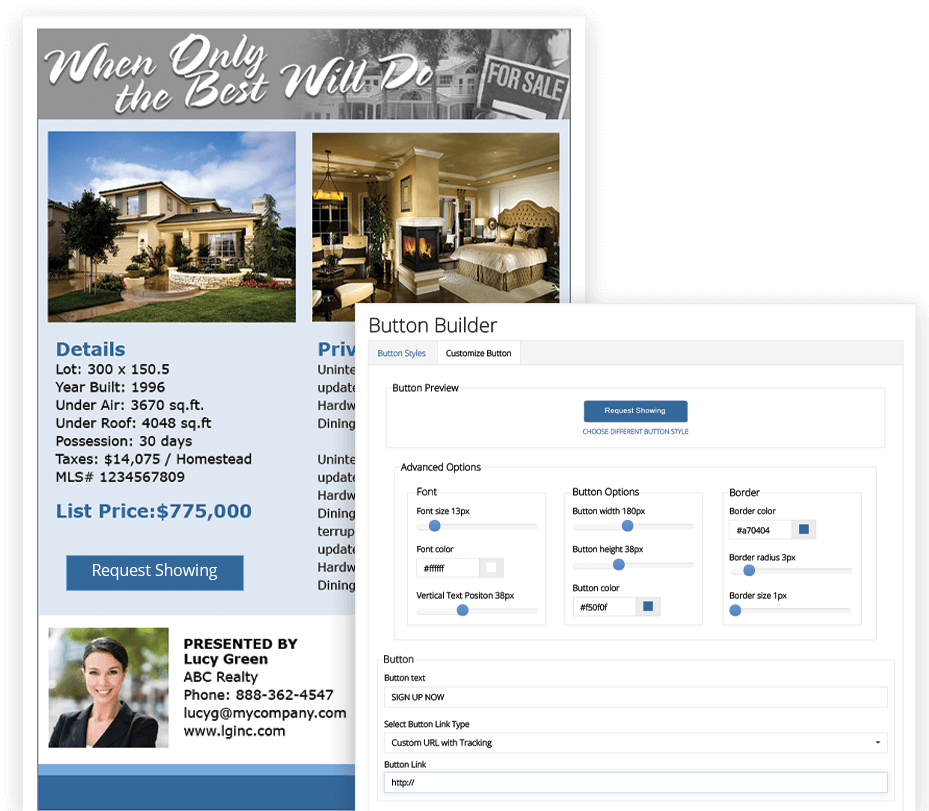**Detailed Caption:**

The image features a comprehensive real estate information layout with distinct sections and color schemes. At the top, there's a clear white background transitioning into a dark section, which might be either black or gray. This area contains text stating, "When only the best will do," accompanied by icons of a house and a 'For Sale' sign.

Below this, the layout transitions into a blue background showcasing a large, luxurious house and a detailed view of one of its bedrooms. Accompanying these images are detailed property specifications: a lot size of 300 by 150.5, built in 1996, offering 3,670 square feet under air and 4,048 square feet under roof, with possession available in 30 days. The listed taxes are $14,075, with a homestead designation, and the MLS list price is $775,000. Additionally, there's an inviting "Request Showing" button.

Near the bottom, a white box features a photo of a professional-looking woman, labeled "Presented by Lucy Green of ABC Realty," along with her contact information.

Further down, the layout is divided into light blue and dark blue sections. Within these sections, a white pop-out box bordered with blue edges holds advanced button customization tools. It includes "Button Builder" functions, with tabs for button styles, customization, and a button preview. There's also a prominent blue "Request Drawing" button and various advanced options for font, button options, borders, and more. Blue toggle buttons are visible for different settings, and the box includes options to sign up, select button type, and link.